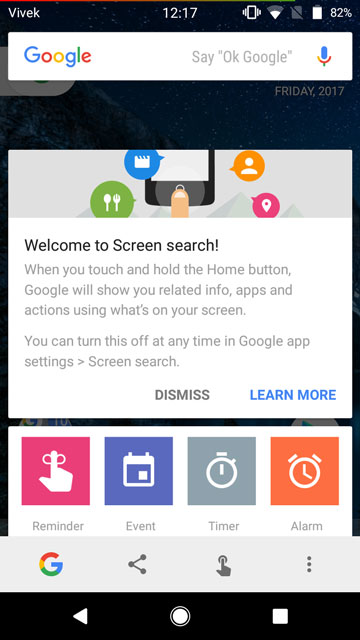The screenshot captures a mobile phone screen with several elements. At the top, the header features white text displaying "Vivec" on the left, "1217" in the center, and five icons on the right side, including a battery icon with a mostly full white bar, positioned second from the right, followed by "82%" in white text at the top-right corner. Below this header, a white rectangular search bar is shown, containing the Google logo on the left and a blue microphone with a multicolored stand icon on the right. Justified to the right side of the search bar is light gray text reading "Say 'OK Google.'"

Further down, a white square pop-up message is displayed. The header of the pop-up includes a cartoon-style image on a light gray background, portraying the bottom of a black mobile phone with a white screen. Around the phone screen, from left to right in an arc, are speech bubble icons with colored backgrounds: green, blue, orange, and pink. Each bubble contains a white icon, respectively showing a spoon and fork, a director's clapboard, a generic profile picture silhouette, and a geolocation pin. Additionally, a cartoon finger is depicted pointing towards the mobile phone. 

Below this image, the pop-up has text on a white background. The top line reads "Welcome to Screen Search" in medium gray text. Beneath it, light gray text explains, "When you touch and hold the home button, Google will show you related info, apps, and actions using what's on your screen." A line break follows, with more light gray text stating, "You can turn this off at any time in Google app settings." Next to this text, an arrow points to "Screen Search." At the bottom-right of the pop-up, medium gray text says "Dismiss," and adjacent to it, blue text reads "Learn More."